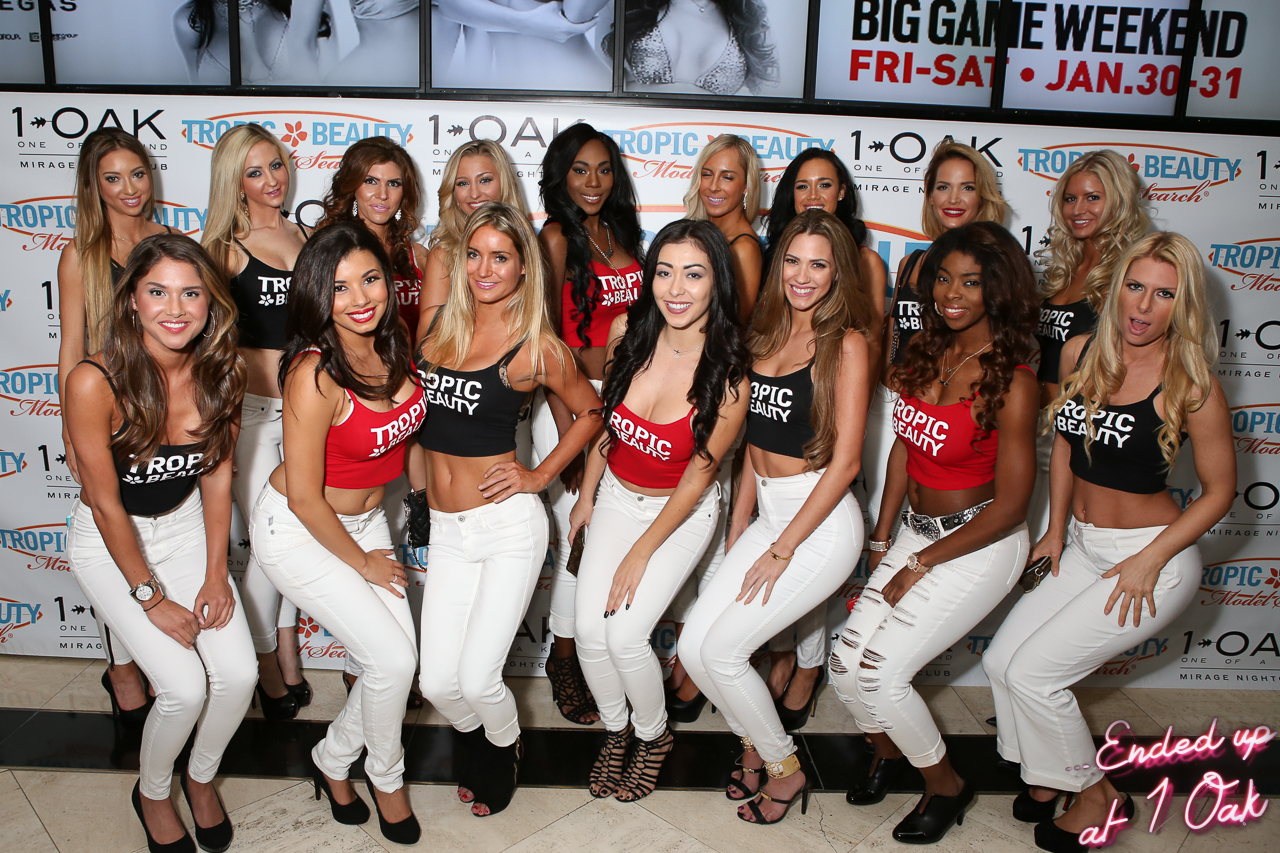In the image, a group of 16 to 17 women of mixed races are posing in two rows against a white backdrop adorned with various advertisements. Prominently displayed behind them is a blue logo for "Tropic Beauty." The backdrop also features black text that reads "Big Game Weekend," red text that announces "Friday to Saturday, January 30 to 31," and an overlay in cursive stating "Ended Up at One Oak" in the bottom right corner. 

The women are dressed uniformly in tight white jeans and high heels of various colors. They alternate between black and red tank tops, all bearing the white text "Tropic Beauty" in all caps. Their hair and makeup look meticulously done, with many sporting long, blonde or brown hair. The front row consists of seven women kneeling or crouching to ensure everyone behind them is visible, while everyone else stands, all smiling directly at the camera. This coordinated and polished look suggests they are part of a promotional event or a photoshoot.